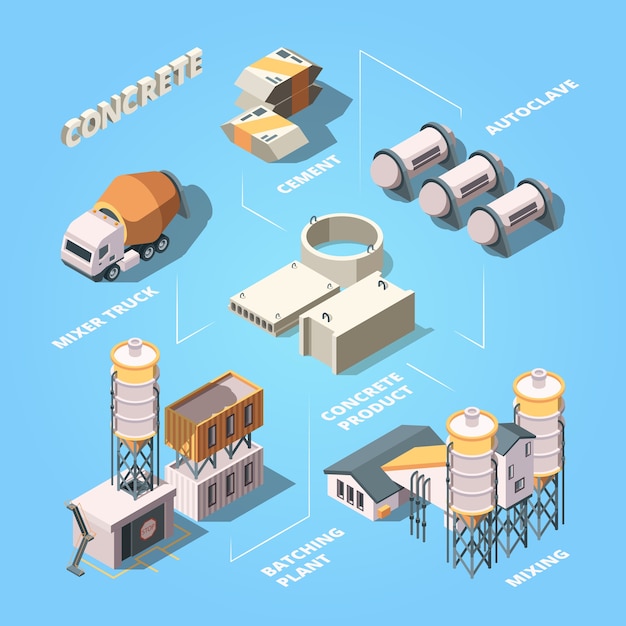The image depicts a detailed illustration of a concrete cement plant set against a pale blue background. Dominating the composition is the batching plant, characterized by a small building or container topped with a tower and labeled clearly in white text. Adjacent to it on the right, two towers are connected to buildings identified as the mixing area. Central to the scene are several gray structures and a circular setup marked as concrete product, illustrating the production phase.

Towards the upper right, there are three canister-like devices labeled autoclave. At the top, structures marked with "cement" indicate the beginning of the cement processing. To the upper left, an illustration of a white and orange cement mixer truck is present beneath the label "mixer truck," reinforcing the focus on transportation within the plant.

The entire plant, including the buildings and equipment, is illustrated in a 3D style with a color palette primarily consisting of white, orange, and yellow. The interconnected processes, highlighted by white lines, depict a systematic workflow of how concrete is mixed, processed, and distributed within the plant.